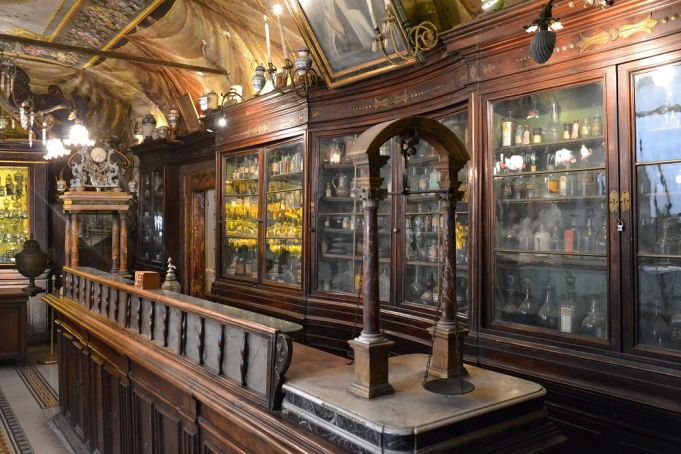The image depicts an ornately decorated, old-style indoor bar that exudes an almost haunted ambiance. The scene appears intentionally designed to look worn and decrepit, perhaps even as set dressing for a venue or an amusement park attraction. The bar features a massive wooden cabinet with glass doors, its shelves filled with dusty bottles of various spirits and liquids, lending to the feeling of abandonment. Draping fabric and carpet-like decorations hang from the concave ceiling, which is adorned with fresco paintings and medieval motifs. The setting is brightly lit, showcasing elaborate details such as a counter with an arch design, numerous candles, and a partitioning element in front of the wall of bookcases in the far back. These bookcases are loaded with bottles and small trinkets, further enhancing the historical and almost fantastical vibe of the space.